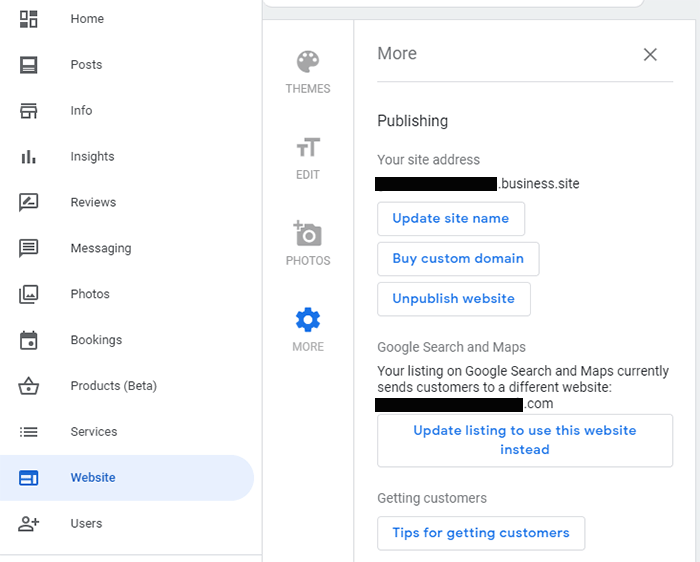This detailed screenshot appears to portray a business website management dashboard. On the left-hand side, there's a vertical toolbar featuring a series of icons and labels:

1. **Home** - Represented by two black and two white squares.
2. **Posts** - Depicted as a piece of paper.
3. **Info** - Icon of a small house.
4. **Insights** - Illustrated by a bar graph.
5. **Reviews** - Shown as a text bubble.
6. **Messaging** - Another text bubble with lines of text.
7. **Photos** - An image emerging from a square.
8. **Bookings** - A calendar page.
9. **Products (Beta)** - A shopping basket icon.
10. **Services** - A bulleted list.
11. **Website** - An icon depicting a website.
12. **Users** - Illustrated by a person's head with a plus.

The interface is currently focused on the "Website" option. Displayed to the right are further customization options:

1. **Themes** - Symbolized by an old painter's palette.
2. **Edit** - A smaller 'T' and a larger 'T'.
3. **Photos** - An old-style camera with a plus on it.
4. **More** - Represented by a cogwheel.

The "More" section is currently selected, offering additional settings:

- **Publishing** - This includes options such as "Your site address: blackedout.business.site" and the ability to "Update site name by custom domain." The website is marked as unpublished.
- **Google Search and Maps** - Noting that the current listing sends customers to "blackedout.com," with an option to update the listing to use the current website.
- **Getting Customers** - Provides tips for acquiring customers.

This dashboard likely belongs to a business website software interface designed for managing and publishing business content, navigating analytics, and optimizing for search listings.